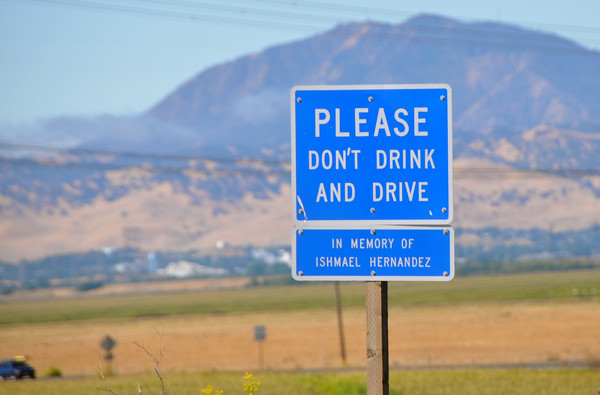In this contemporary photograph, a serene blue sky stretches across the background, framing a distant mountain range. Electrical wires span the scene, crossing the hazy expanse where the mountains meet a vast plain. Below, clustered houses are faintly visible, their outlines softened by the distance. The foreground transitions into verdant pastures and sunlit prairies, intersected by a paved road that winds through the landscape. On the left-hand side at the bottom of the image, a blue SUV travels along this road, moving towards the right. Two small, indistinct signs sit beside the road, hinting at messages unreadable due to the distance. Prominently in the foreground, a blue sign with white lettering stands as a poignant reminder: "Please Don't Drink and Drive." Beneath it, a smaller sign carries a heartfelt memorial: "In Memory of Ishmael Hernandez."